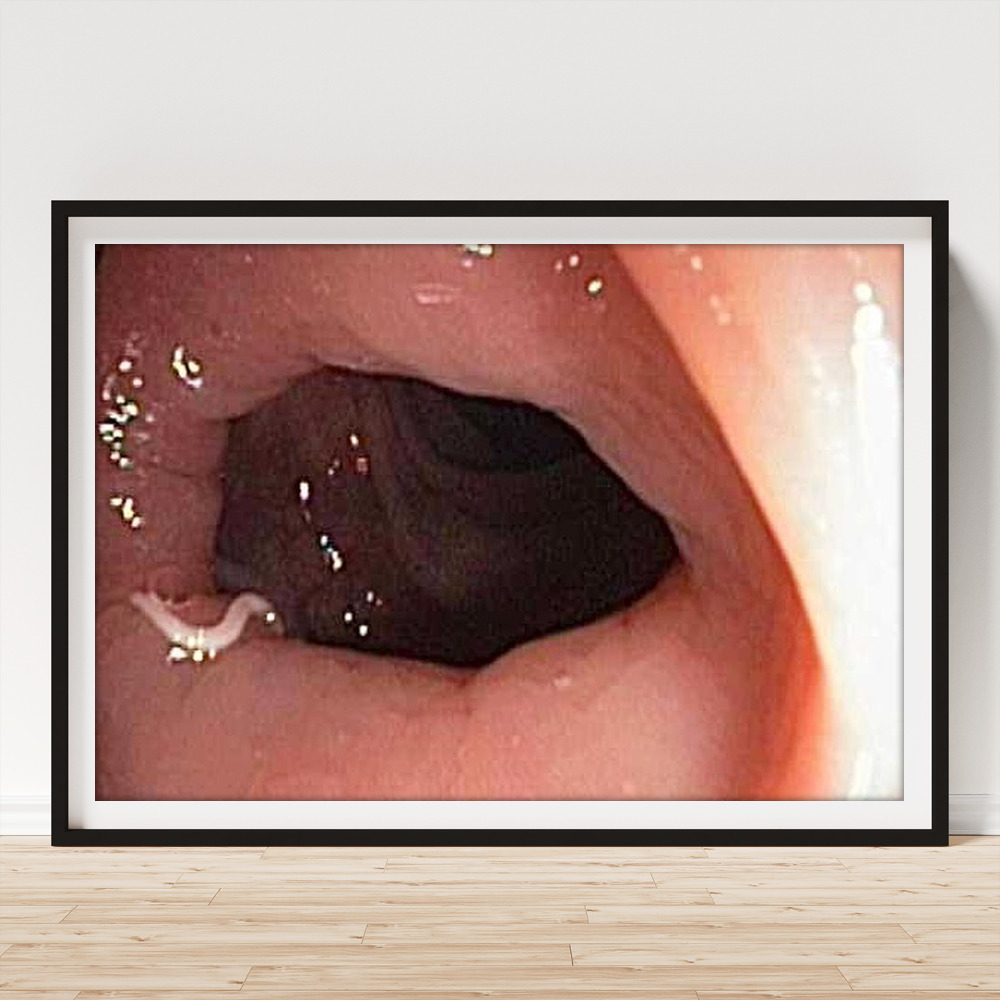This photograph captures a horizontally framed image propped against a white wall and a light wood-grained floor. The composition includes a black frame with a white matting surrounding the picture. The focal point of the image appears to be an anatomical representation, resembling the interior of a human colon. The central portion of the picture shows a dark tunnel or hole, bordered by pink, shiny flesh. Bright light reflects off the right side of the image, revealing a moist, vein-riddled surface. A distinctive, small, white, sliver-like structure emerges from the lower left of the darkened hole, resembling a worm or defect, adding a stark contrast against the surrounding tissues.